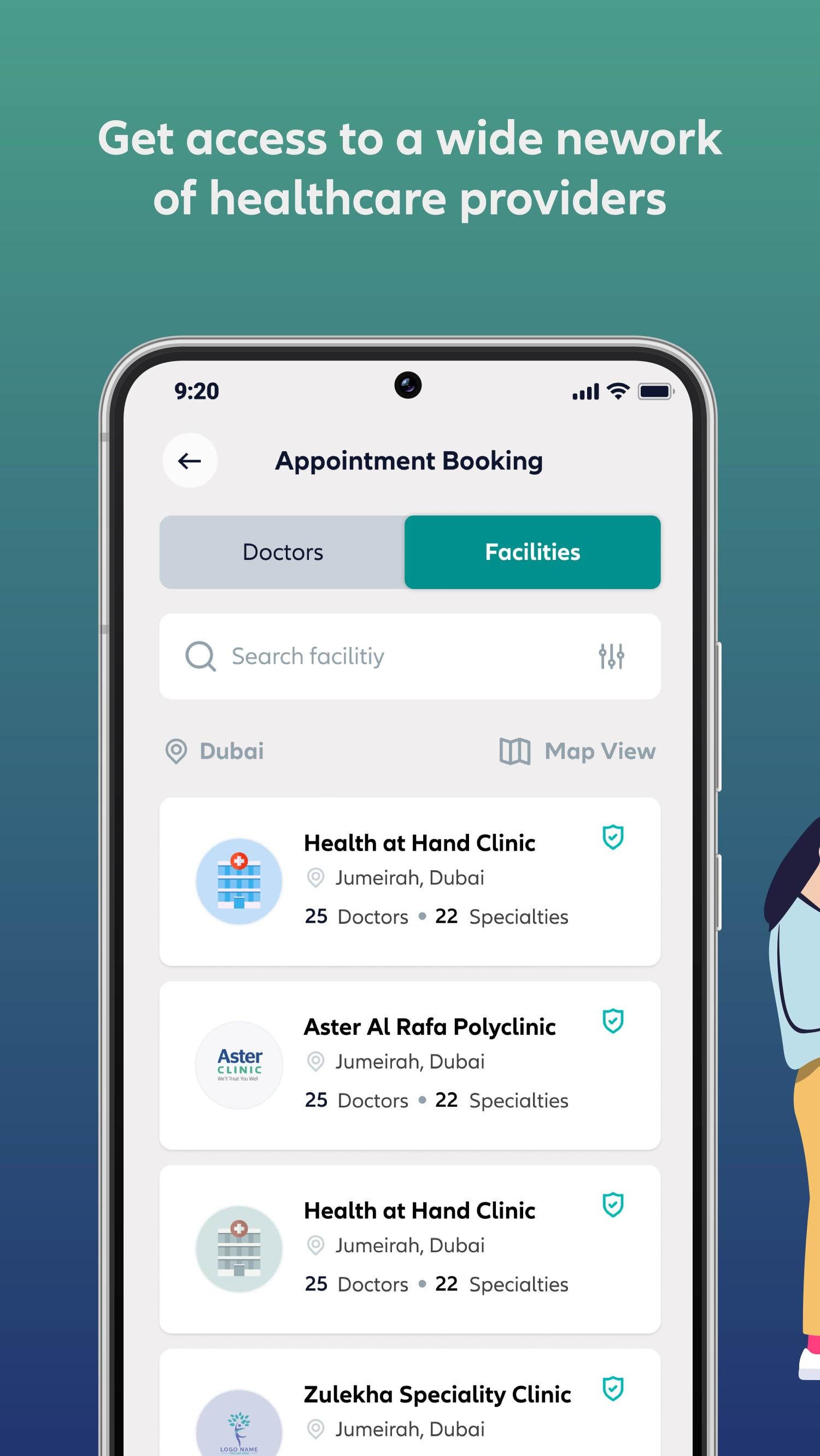The image is an advertisement for a healthcare provider's website or app, designed in a rectangular format that is taller than it is wide. The background features a gradient that begins with a turquoise green at the top and transitions into a darker, purplish-blue hue at the bottom. In the center of the advertisement is a graphic of a smartphone displaying the website or app interface. 

At the top of the smartphone screen, the title "Appointment Booking" is prominently displayed in black text. Below this title, there are two distinct buttons. The left button has a light gray background with the word "Doctors" in black text. The right button features the teal green color again, with "Facilities" written in white text.

Beneath these buttons is a white, rectangular search bar with light gray text that reads "Search facility." To the left of this text, there's an icon of a magnifying glass. Further down the screen is a list of different health clinics, each presented in a rectangular box with a white background and black text. Each clinic name is accompanied by a circular icon located to the left of the name.